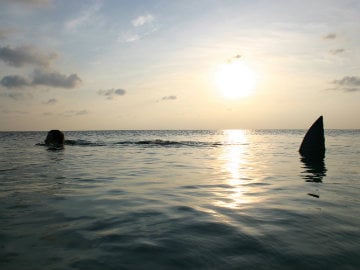The photograph captures a serene ocean scene at either sunset or sunrise, with muted, unsaturated colors dominating the composition. The sky showcases a gradient of blues and grays, sprinkled with pale white and gray fluffy clouds. Near the horizon, the sun's proximity adds a subtle hint of yellow and light pink to the scene, casting its reflection on the water below. The ocean itself transitions from a dark, almost bluish-gray hue to lighter shades where the sun’s reflection touches. On the right side of the image, a shape resembling a fin—possibly from a shark or dolphin—breaks the surface of the water, adding an element of mystery. Meanwhile, on the left, a somewhat spherical dark shape emerges, which might be a human head or another unidentified object. Additionally, a lone sailboat with only its dark sail visible is situated to the right of the image. A small stretch of land or a large rock lies just ahead of it, contributing to the tranquil yet enigmatic atmosphere of the scene. The water around the sun glistens in shades of white and pink, capturing the fleeting beauty of this transitional time of day.